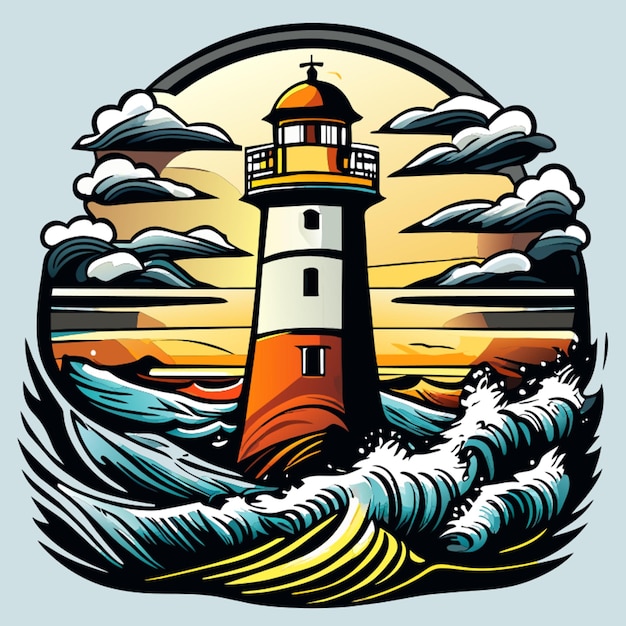This detailed digital drawing, potentially computer-generated, features a prominently centered lighthouse encircled by a large black border. The lighthouse itself stands resiliently over choppy blue waves adorned with foamy white caps, reflecting a tumultuous sea. The lighthouse’s base is characterized by an orange, and rust hue with a black window, transitioning to two white sections with black windows. The top includes a circular balcony and an orange domed roof crowned with a cross-like figure.

The background is a mesmerizing fusion of pale blue transitioning into a vivid sunset gradient of orange and yellow, lending an ethereal glow to the scene. Fluffy white and grey clouds creep into the circle, blending into the sunset hues. The interplay of colors—gray, black, blue, and golden yellows—creates a dynamic and atmospheric setting, accentuating the lighthouse's steadfastness amidst the vibrant seascape.